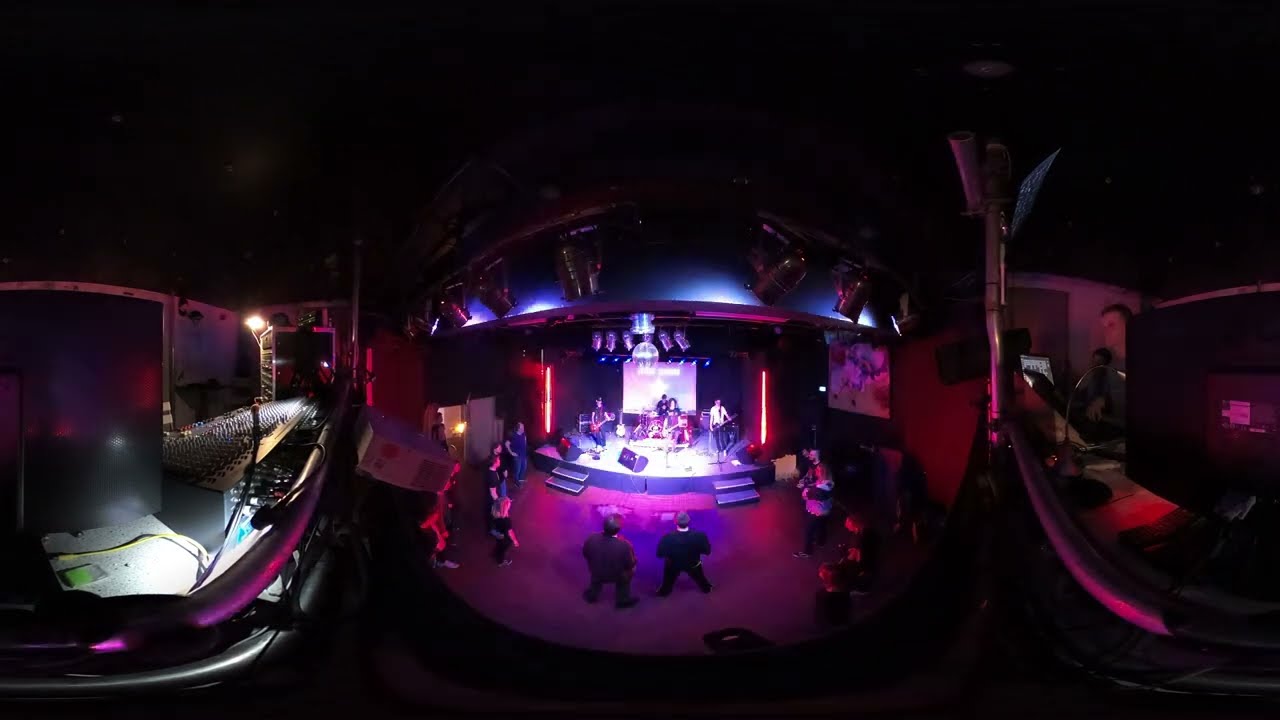The image captures the interior of a dimly-lit night venue during a live music performance. Dominating the scene is a stage bathed in purple-violet lighting, where a four-member band is actively performing. The band consists of what looks like a drummer positioned at the back, two guitarists, and a bassist. To the left of the image, a mixing desk and some technical equipment are visible, while two computer monitors and a microphone stand can be seen on the right. A man, possibly a crew member, is situated near these devices, suggesting he may be in charge of sound or recording duties. Above the stage, a mirror ball hangs, adding a touch of classic venue decor. There is also a screen behind the band, displaying their name, though it is illegible from this angle. The sparse audience, composed of around 13 individuals, stands rather than sits, indicating an intimate gig setting. The overall ambiance combines darkness in the surrounding area with concentrated, vibrant lighting focused on the performers, making the stage the central focal point in the otherwise shadowy room.